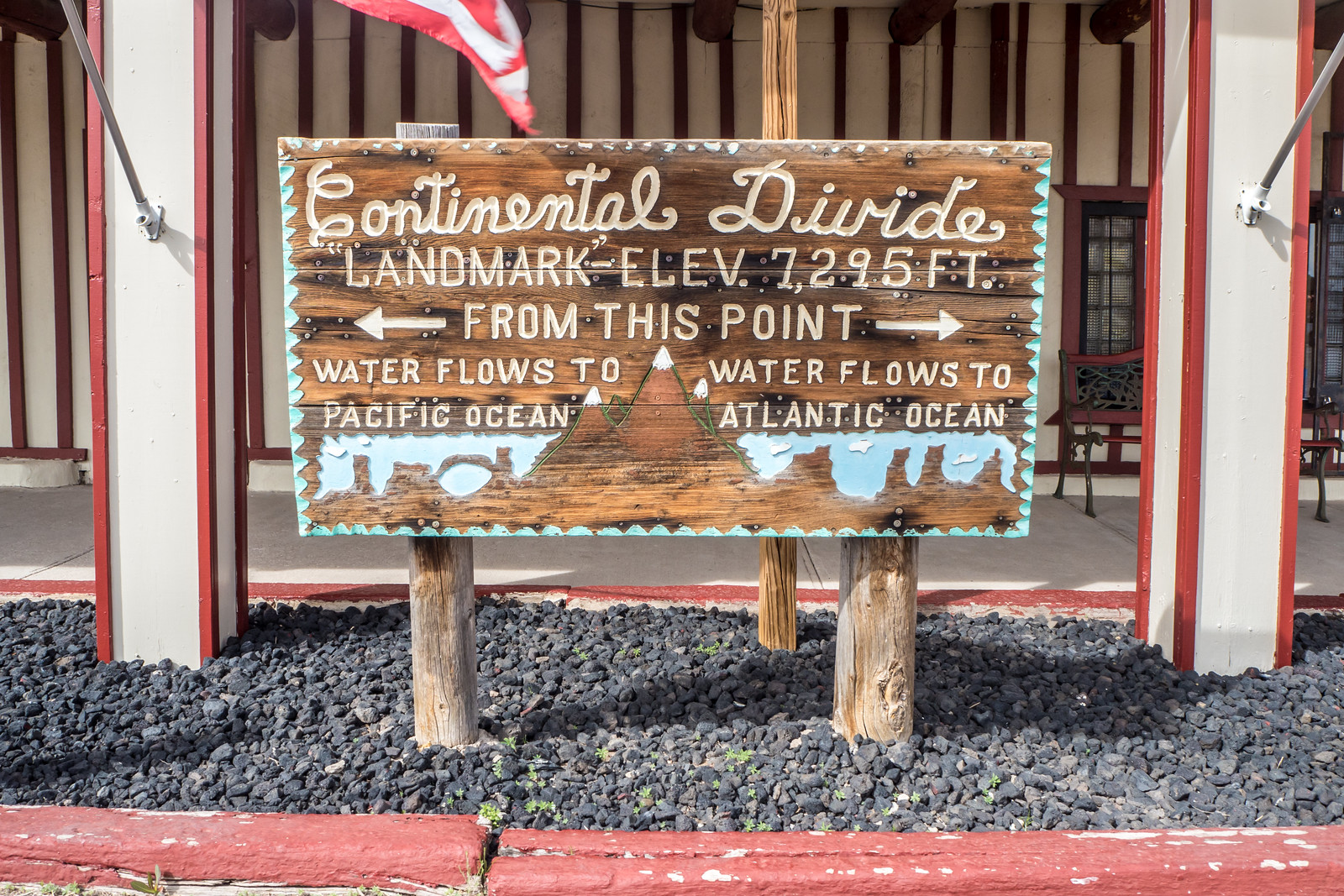A detailed wooden sign, mounted on two sturdy wooden posts, stands outside a white and red-painted building, likely a store or hotel. This building, adorned with benches, windows, and flags on its red-trimmed columns, serves as a backdrop for the sign, which is set within a gravel area surrounded by a red curve.

The sign itself is intricately detailed, reading "Continental Divide Landmark Elevation 7295 feet" in cursive white text. Below this, in capital letters, it states, "FROM THIS POINT," with arrows pointing left and right. The left arrow indicates that "Water flows to the Pacific Ocean," while the right arrow notes that "Water flows to the Atlantic Ocean." 

In the middle of the sign, there is an artistic rendition of mountain peaks painted white, flanked by two bodies of blue-painted water, representing the two oceans, with visible landmasses and stone pillars beneath the water surface. This visual depiction illustrates the water flow directions specified by the arrows.